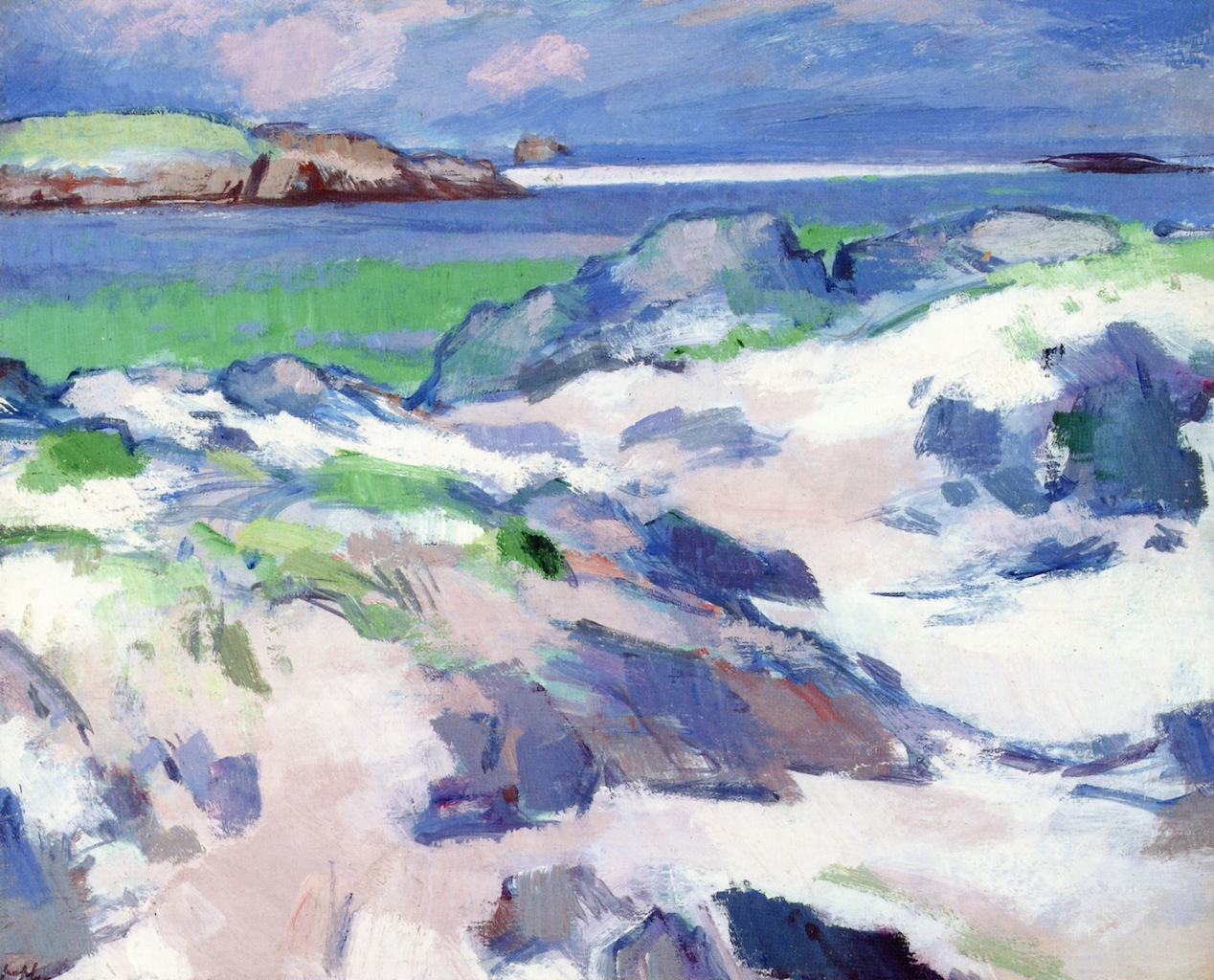The image captures a highly abstract, mixed-media painting of a seaside landscape rendered in varying tones of greens, blues, and whites. In the foreground, a quarter up from the bottom, the artist has textured the canvas to resemble a shoreline with smooth, brown and gray rocks, some of which are partially submerged in the water. The seascape here is vibrant with blue and green hues featuring small white caps on the waves. 

Moving upward, the left side reveals a grassy outcropping rendered in a rich green, adding a natural contrast to the rocky shore. Extending from this outcropping into the water is a brown jetty, suggestive of a rocky pier, creating a focal point with its sturdy appearance.

Above these elements, the open water stretches out in shades of flat blue, indicative of a calm sea. There is also a subtle suggestion of something dark in the water, accompanied by a plume of white, hinting at a boat or an animal moving through. 

In the distant background, the dark blue sky is speckled with puffy clouds in varying shades of blue and white, providing a dramatic and calming backdrop to this coastal scene. The entire composition, with its loose brushstrokes and abstract forms, captures the serene yet dynamic nature of the seaside.